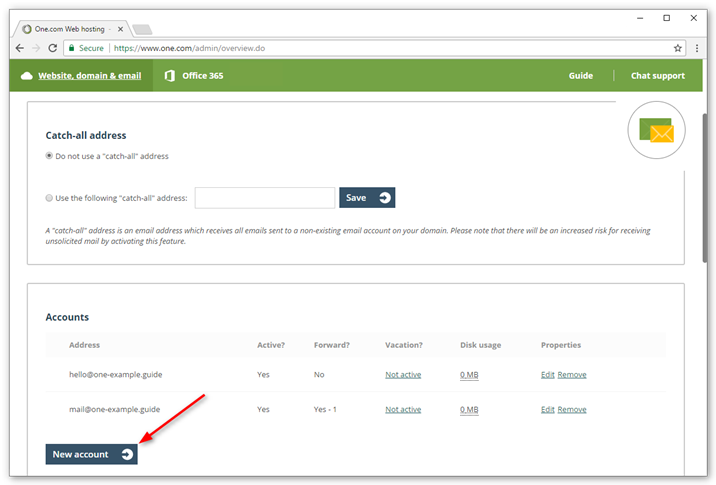Caption: The image depicts a screenshot of the One.com web hosting interface, specifically the overview page (URL: one.com/overview.do). The page is secured with a green lock icon visible in the browser's address bar. 

Directly below the address bar is a bright olive green ribbon with white text. On the left side, the ribbon displays "Website Domain and Email," followed by "Office 365" in the center, and "Guide" on the right side. Adjacent to "Guide," there's an option for "Chat Support."

Under this ribbon, there's a gray line, beneath which the text reads "Catch all addresses. Do not use a 'catch-all' address. Use the following 'catch-all' address:" An input field is provided for the address, accompanied by a teal button labeled "Save" in white text.

At the bottom of the screen, there is a teal button with white text labeled "New Account" on the left side, highlighted with a red arrow pointing towards it. This button is likely intended for educational purposes to assist users in starting a new account.